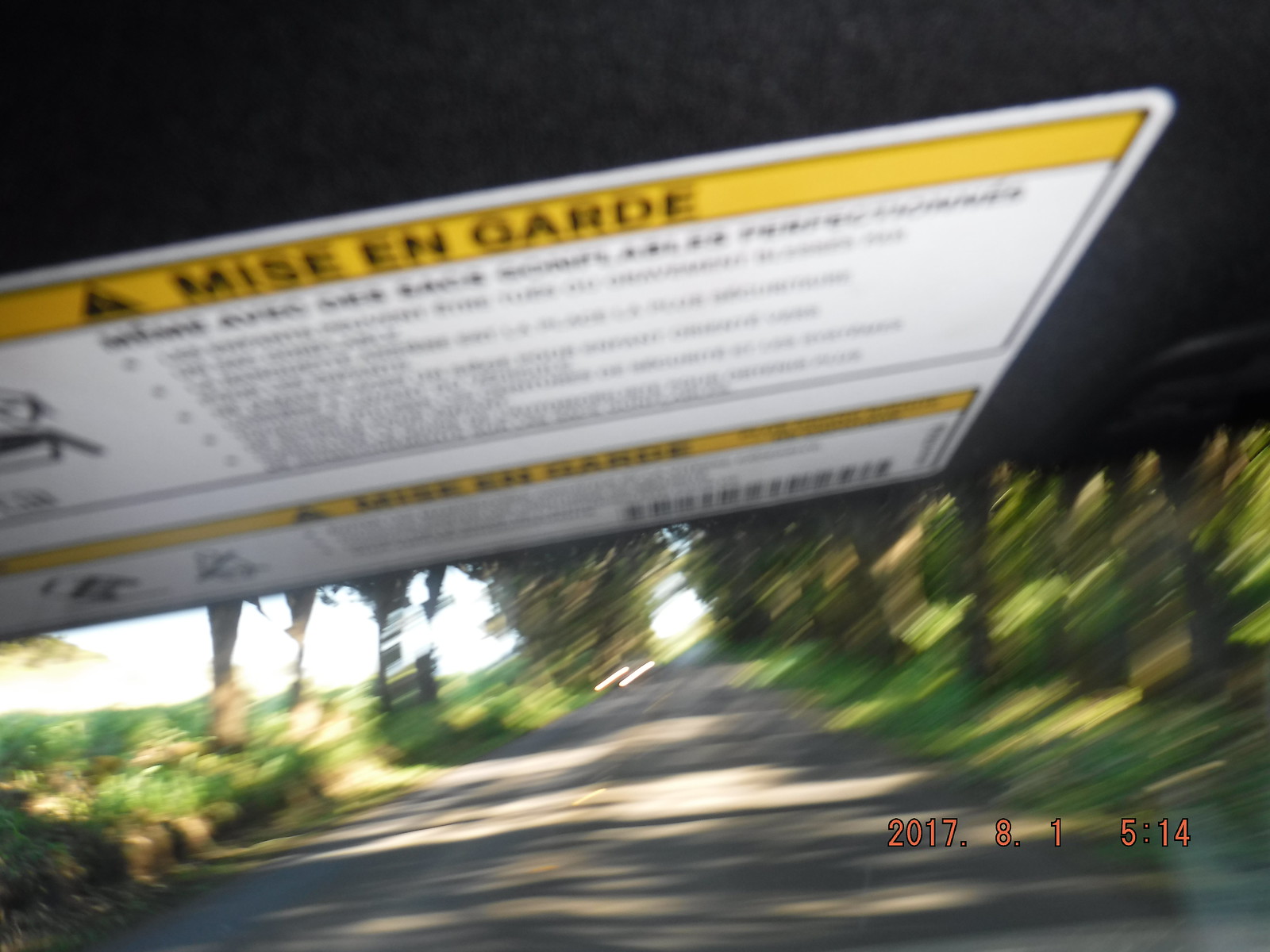This color photograph, taken outdoors during daylight on August 1st, 2017, at 5:14 PM, captures a blurry scene likely shot from inside a moving car, possibly through the windshield. The image prominently features a roadway flanked by palm trees with some sunlight filtering through their leaves, set against a clear sky. The perspective suggests traveling through an overpass or tunnel. Mounted high to the interior ceiling of the car, a white and yellow warning sign reading "Meisingard" in a non-English language is visible above the road. The photograph also shows the vague blur of green foliage and tree trunks along the road and distant blurry headlights, indicating oncoming traffic.